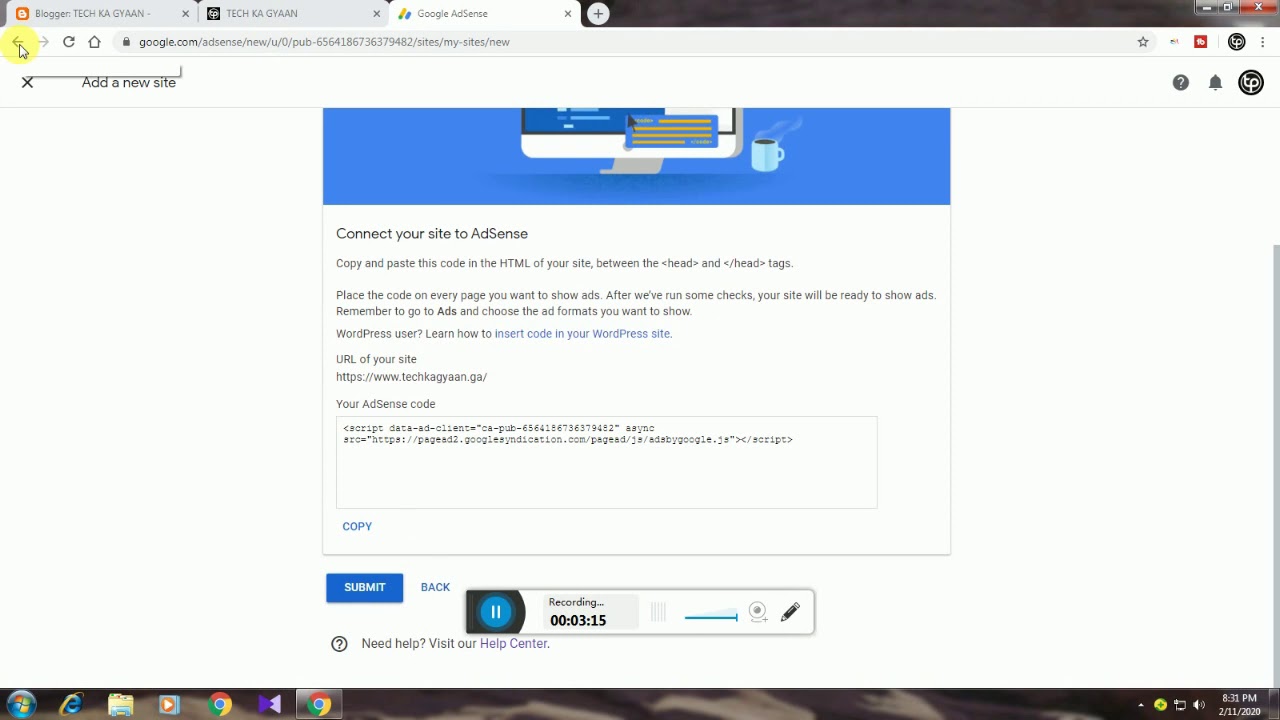This screenshot captures a detailed view of a desktop featuring the Google Chrome web browser with three open tabs. The first tab is a Blogger page, the second tab is titled "Tech Kyagyan," and the currently active third tab is open to the Google AdSense website. On the active AdSense tab, the mouse cursor hovers over the back arrow on the top browser menu, which is highlighted in yellow. 

The browser's top menu bar includes the back and forward navigation arrows, a refresh button, a home button, the URL bar displaying the AdSense page address, an empty star icon indicating the site is not bookmarked, and a few extension icons. Among the extensions, one displays some text, while the others are represented by a red box and a black circle. Positioned to the far right of the menu bar are the three vertical dots opening Chrome's main menu.

On the webpage itself, a blue banner featuring a graphic of a coffee cup is prominently displayed at the top. Below the banner, instructions guide the user on how to connect their site to AdSense, accompanied by a rectangular box containing the AdSense code. Directly beneath the code box is a blue link for copying the code. At the bottom of the instructions are two buttons: a blue-highlighted "Submit" button and a non-highlighted "Back" button. A notification at the bottom of the window indicates that the session is currently being recorded.